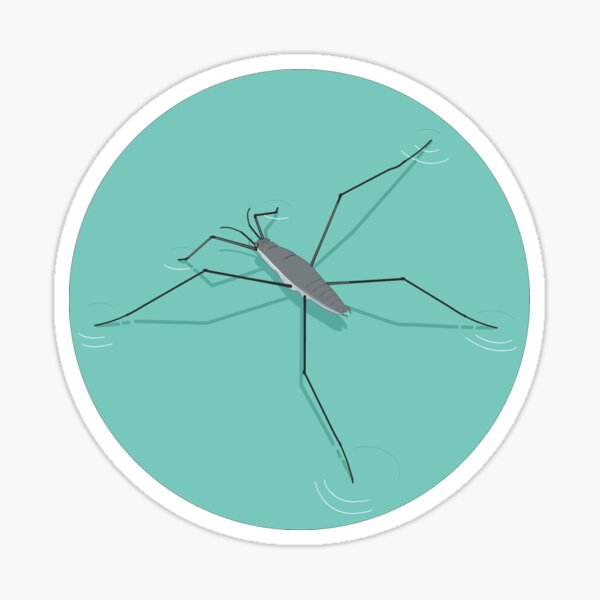In the center of a light beige background sits a detailed digital rendering of a water strider depicted in a circular icon. The icon features an aqua-colored center, representing the surface of water, bordered by a white circle with a slight drop shadow. The water strider has a gray oblong body with grayish-black legs and two antennae that curve towards its head. It is illustrated in a cartoon-like manner. The insect has four long legs, positioned two on either side of its body, and two shorter legs near its head. The strider creates small white ripples at the point where each of its legs meets the water's surface, further emphasizing its ability to walk on water without sinking. The image combines elements of realism and abstraction to effectively convey the water strider's unique locomotion.